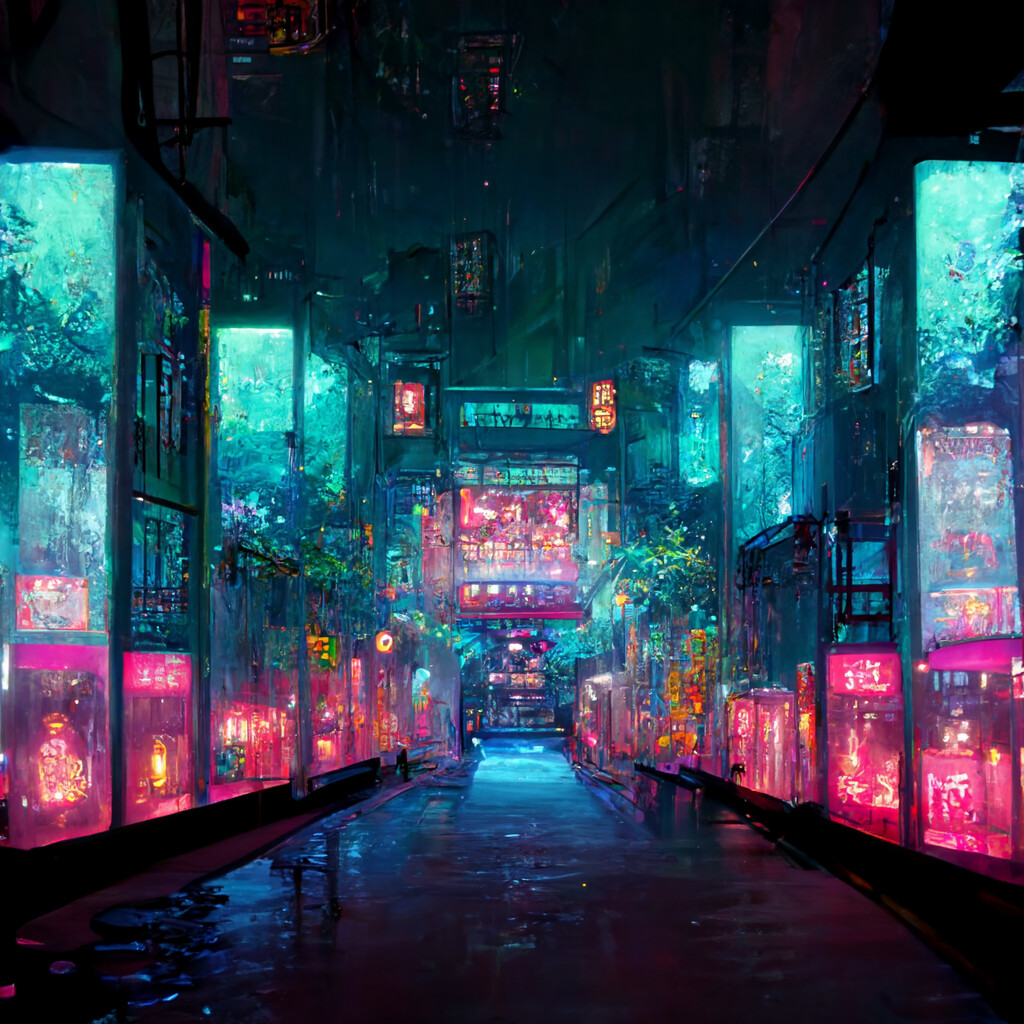The image depicts a highly detailed, watercolor painting of a futuristic, cyberpunk-style city street at night. The street, which resembles an alley or a walkway, appears wet and reflective, suggesting it may be covered in water, adding a shimmering effect. On both sides of the street, there are symmetrical rows of buildings with green tops and vibrant, hot-pink illuminated storefronts. These buildings feature several inscriptions and are adorned with glowing neon blue glass on the upper stories, creating a stark contrast with the pink lighting below. The scene is richly lit from within the buildings, which display amber-colored lamps and possible plant life, adding a sense of lushness to the urban environment. In the middle of the composition, there is a large store-like building, leading to a bridge further down, which connects to additional upper stories. In the far distance, a towering structure looms, adorned with a large, glowing window in hot pink and neon blue accents. The overall scene captures a blend of urban aesthetic and futuristic elements, making it a captivating representation of a vibrant, yet dystopian cityscape.